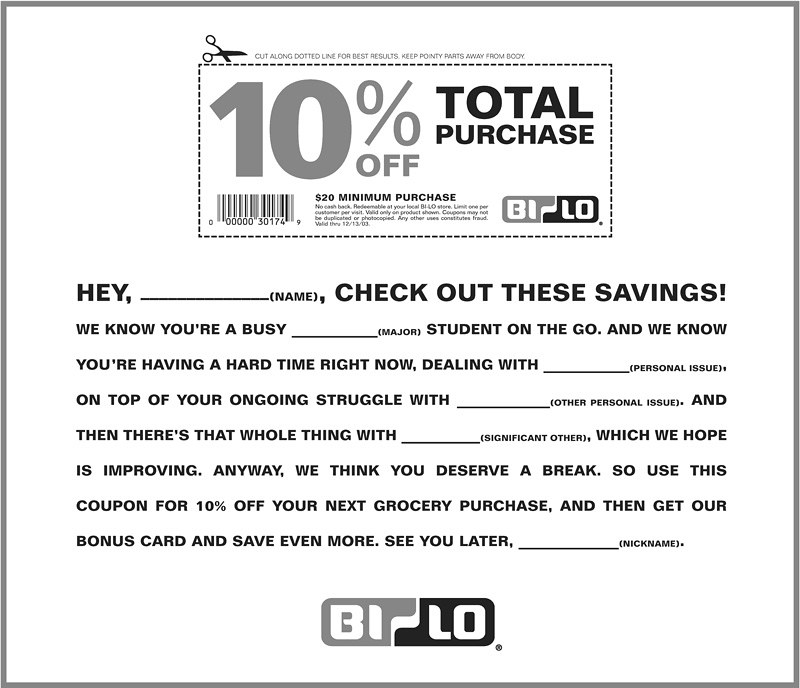The image displays an advertisement featuring a coupon offering 10% off a total purchase with a minimum spend of $20. The number "10%" is rendered in gray, while "total purchase" is in black. The coupon is enclosed within a dotted rectangle with a scissors icon, indicating it should be cut out. Below the coupon is a personalized message: "Hey [Name], check out these savings! We know you're a busy [Major] student on the go, and we know you're having a hard time right now dealing with [Personal Issue] on top of your ongoing struggle with [Other Personal Issue]. And then there's that whole thing with [Significant Other], which we hope is improving. Anyway, we think you deserve a break, so use this coupon for 10% off your next grocery purchase, and then get our bonus card to save even more. See you later, [Nickname]." The text includes placeholders for the recipient to fill in their details, adding a personalized touch. The Bilo logo appears at the top and bottom center of the advertisement, emphasizing the brand.